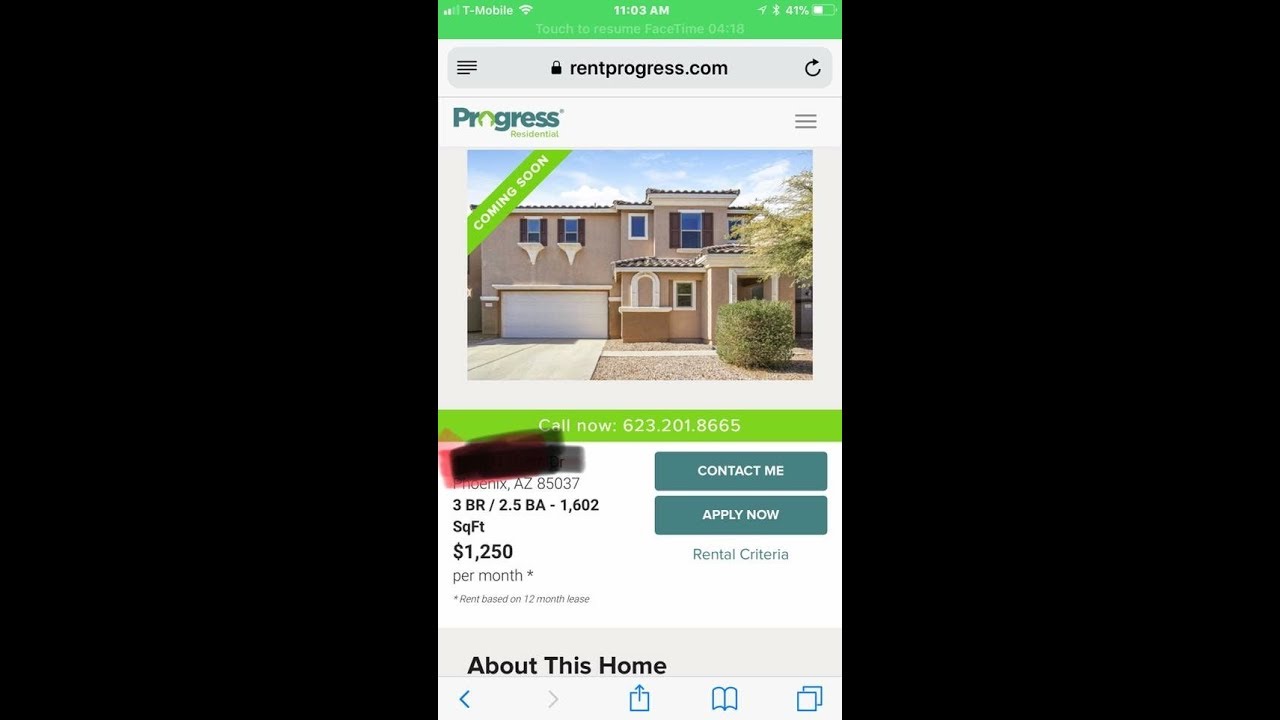This image, sourced from the rentprogress.com mobile website, features a sleek design with a green theme. At the top of the screen, there is a green strip displaying typical mobile elements such as the time (11:50 AM), battery life, and connectivity status, possibly indicating a T-Mobile network.

Below this, the website's branding is showcased in a gray bar bearing the text "rentprogress.com." Directly underneath, the word "Progress" is prominently displayed, with a unique color scheme where the letter "O" is in lime green and the remaining letters are in blue. 

The main focus of the image is a high-quality photograph of a charming house accompanied by the text "COMING SOON" in a lime green banner located in the upper left-hand corner. Additionally, there is a lime green strip adjacent to the photo, which includes a call to action with a phone number. The house's address is censored for privacy, showing only that it is located in Phoenix, Arizona.

Details about the property state it is a three-bedroom, two-and-a-half-bath home with 1,600 square feet, available for a monthly rate of $1,250. To the right of the photo, there are two green buttons labeled "Contact Me" and "Apply Now," inviting potential renters to take immediate action. There is also a section titled "Rent Criteria" in green, which can be clicked to review the requirements for renting the property.